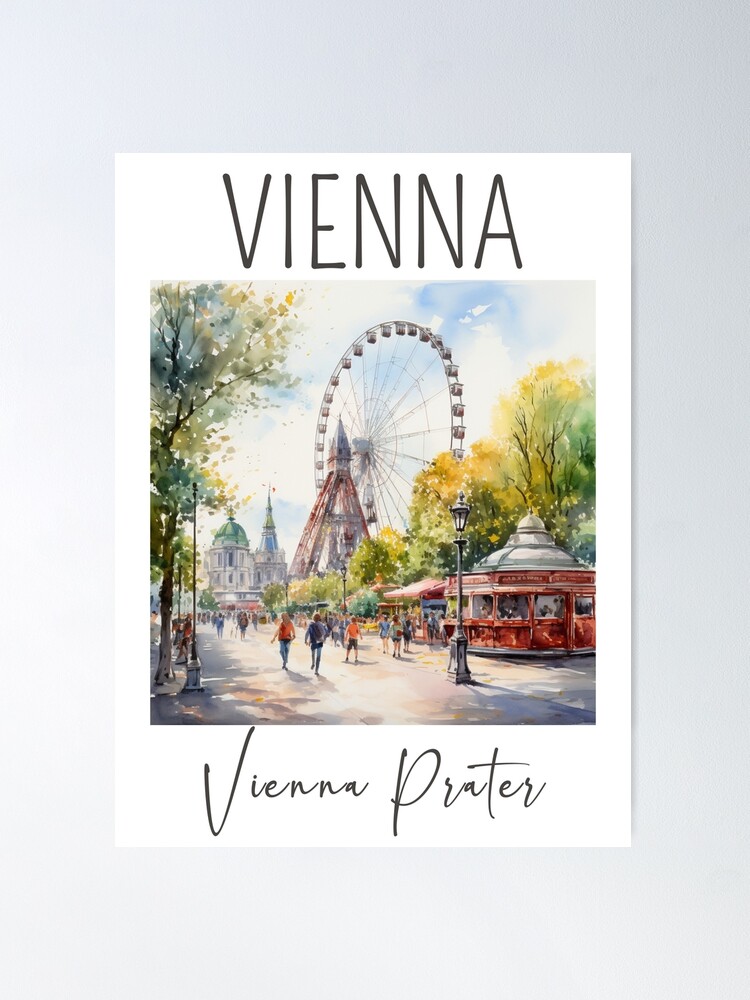The postcard-styled illustration entitled "Vienna" displays a lively outdoor scene possibly set in the famous Vienna Prater. The title "Vienna" is prominently written in capital letters at the top, with "Vienna Prater" inscribed in cursive at the bottom. The artwork, reminiscent of a watercolor painting or possibly an ink drawing with color, showcases a sunny, partly cloudy day. Central to the image is a large Ferris wheel partially obscured by trees. A red-roofed, circular pavilion or carousel stands prominently in the foreground. Surrounding the Ferris wheel, a vibrant fair scene unfolds with people milling about, suggesting a carnival or street fair atmosphere. On the left, a streetlight punctuates the scene, while various buildings including a church-like structure with a dome, and another pyramid-shaped building, complete the backdrop. The light, delicate colors of the trees and structures contribute to a cheerful and picturesque setting.